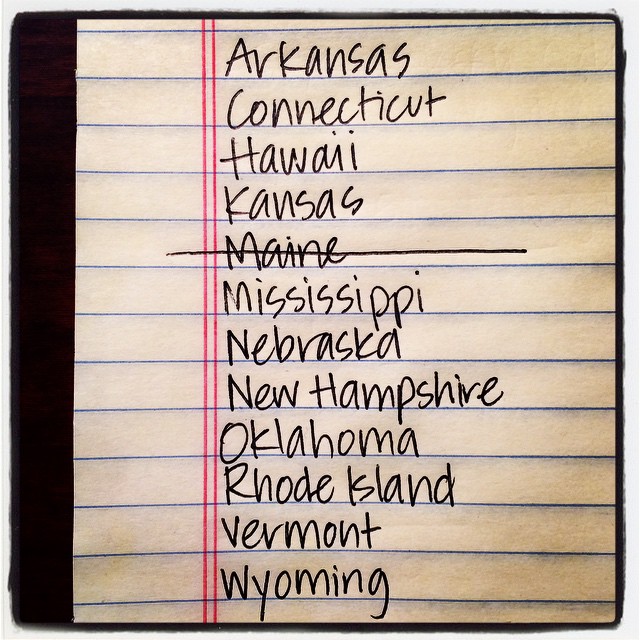The image depicts a mildly stained and faded cut-out section of college-ruled paper, placed over a black background. The paper features horizontal blue lines and two vertical red lines forming a left margin. The names of various U.S. states are hand-printed in black ink, written in alphabetical order. The list begins with "Arkansas" at the top, followed by "Connecticut," "Hawaii," "Kansas," and continues with "Mississippi," "Nebraska," "New Hampshire," "Oklahoma," "Rhode Island," "Vermont," and ends with "Wyoming" at the bottom. Notably, the state "Maine" appears with a horizontal black line crossing it out. All names start with an uppercase letter followed by lowercase letters, and are aligned to the right of the red margin lines.